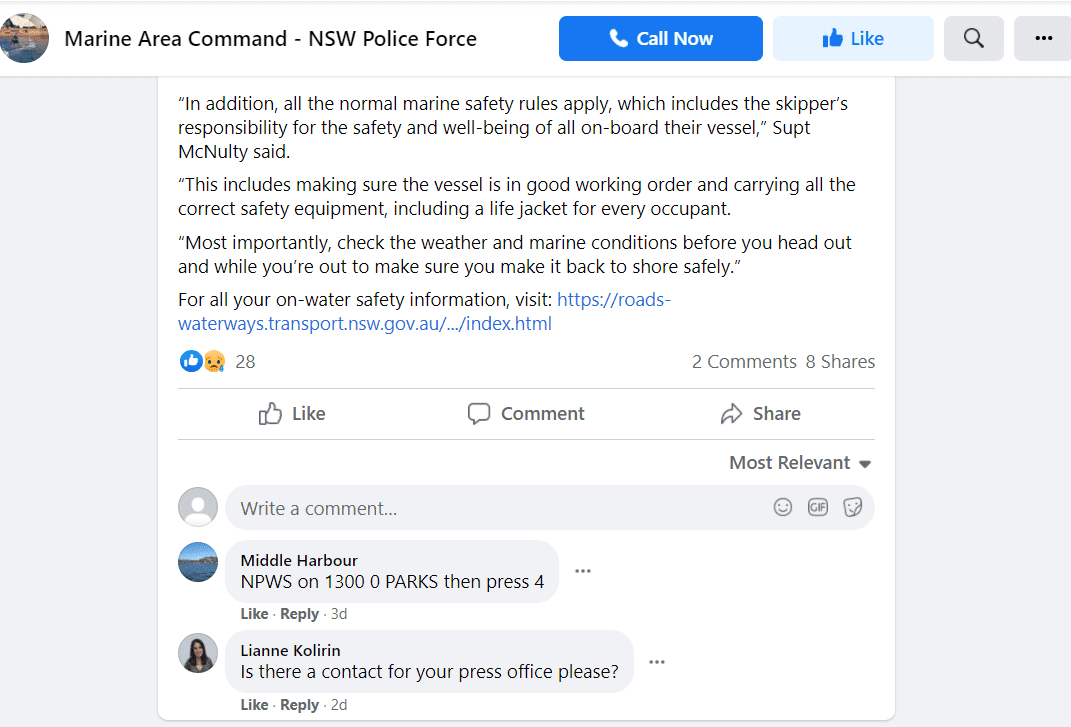Here is your cleaned-up and detailed caption:

---

The screenshot features a light gray background with a white banner running horizontally across the top. On the left side of the banner is a profile icon labeled "Like." To its right, the text "Marine Area Command - NSW Police Force" is displayed in black. Adjacent to this text is a blue "Call Now" button with a phone icon to its left. 

On the right side of the banner, there is a light blue "Like" button featuring a thumb icon, followed by two gray squares. The first gray square contains a magnifying glass icon, and the second one shows the three-dot ellipsis symbol. 

Below the banner, within the light gray background, a central white square displays black text quotes: "In addition, all the normal marine safety rules apply, which includes the skipper's responsibility for the safety and well-being of all on board their vessel," SUPT McNulty said.

The text continues: "This includes making sure the vessel is in good working order and carrying all the correct safety equipment, including a lifejacket for every occupant."

The next paragraph reads: "Most importantly, check the weather and marine conditions before you head out and while you're out to make sure you make it back to shore safely."

The final paragraph states: "For all your on-water safety information, visit: [link to Roads Waterways Transport website]"

Below this text are the icons for "Like" and "Sadness" on the left. On the right, it shows "2 Comments" and "8 Shares." Beneath this section, there is a bar with options to "Like," "Comment," and "Share."

Further below are gray comment bubbles featuring profile icons to the left.